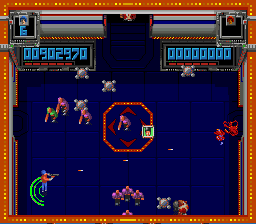This image, slightly wider than it is tall, captures the vibrant essence of a 1980s-style arcade game. The scene is framed by an orange marquee, adorned with clusters of four ascendingly bright orange dots. Inside, the floor is depicted with blue tiles, while foreshortened gray walls define the room's perimeters on the left, right, and top.

At the center of the image, a stop-sign-shaped octagon, bordered with red arrows, possibly serves as a focal point or target. Surrounding this central element are various characters; notably, one character in the lower left corner is armed with a gun and encircled by green, concentric semicircles facing left. This could likely be the protagonist of the game. Additionally, an array of potential monsters or adversaries are scattered throughout the room, adding to the dynamic and engaging atmosphere of the portrayed arcade game.